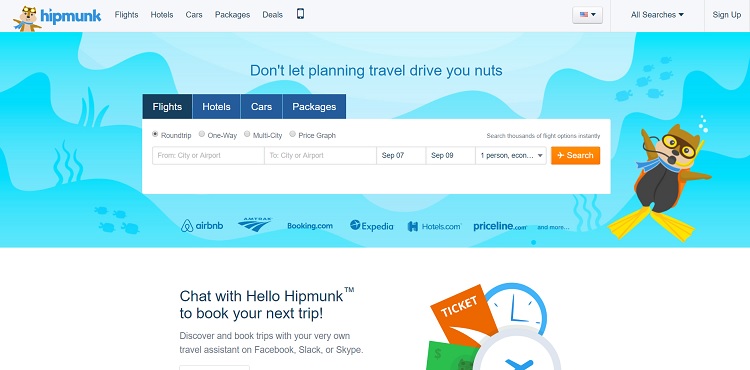**Caption:**
This vibrant, detailed illustration promotes Hipmunk, a travel booking website. In the top left corner, the iconic Hipmunk mascot, a cheerful squirrel, is featured, symbolizing the site's user-friendly travel search options for flights, hotels, cars, packages, and deals. The American flag, labeled "Dr. Mean," is positioned nearby, along with tags for "All Searches" and "Senate."

The background is a captivating underwater scene with seaweed and various fish, adding a whimsical element to the overall design. To the far right, another squirrel appears, this time alongside a yellow fin and a wetsuit, enhancing the aquatic theme. The left side of the image emphasizes Hipmunk's quirky slogan, "Don’t Let Punny Travel Drive You Nuts."

Below this slogan are different travel options: round trip, one way, and multi-city. The booking form suggests a trip from one city airport to another, with sample dates of September 7th to September 9th, for one person, concluding with a prompt to "search thousands" of options.

Logos of popular travel services such as Airbnb, Amtrak, Booking.com, Expedia, Hotels.com, and Priceline are also displayed, highlighting the breadth of comparison options available on Hipmunk. An invitation to chat with "Hello Hipmunk" for personalized trip booking assistance via Facebook, Slack, or Skype is prominently featured.

Additional visual elements include an orange ticket, green cash symbol, and two colorful clocks, contributing to the dynamic and engaging layout of the advertisement. This detailed depiction clearly positions Hipmunk as a comprehensive, fun, and efficient travel booking platform.